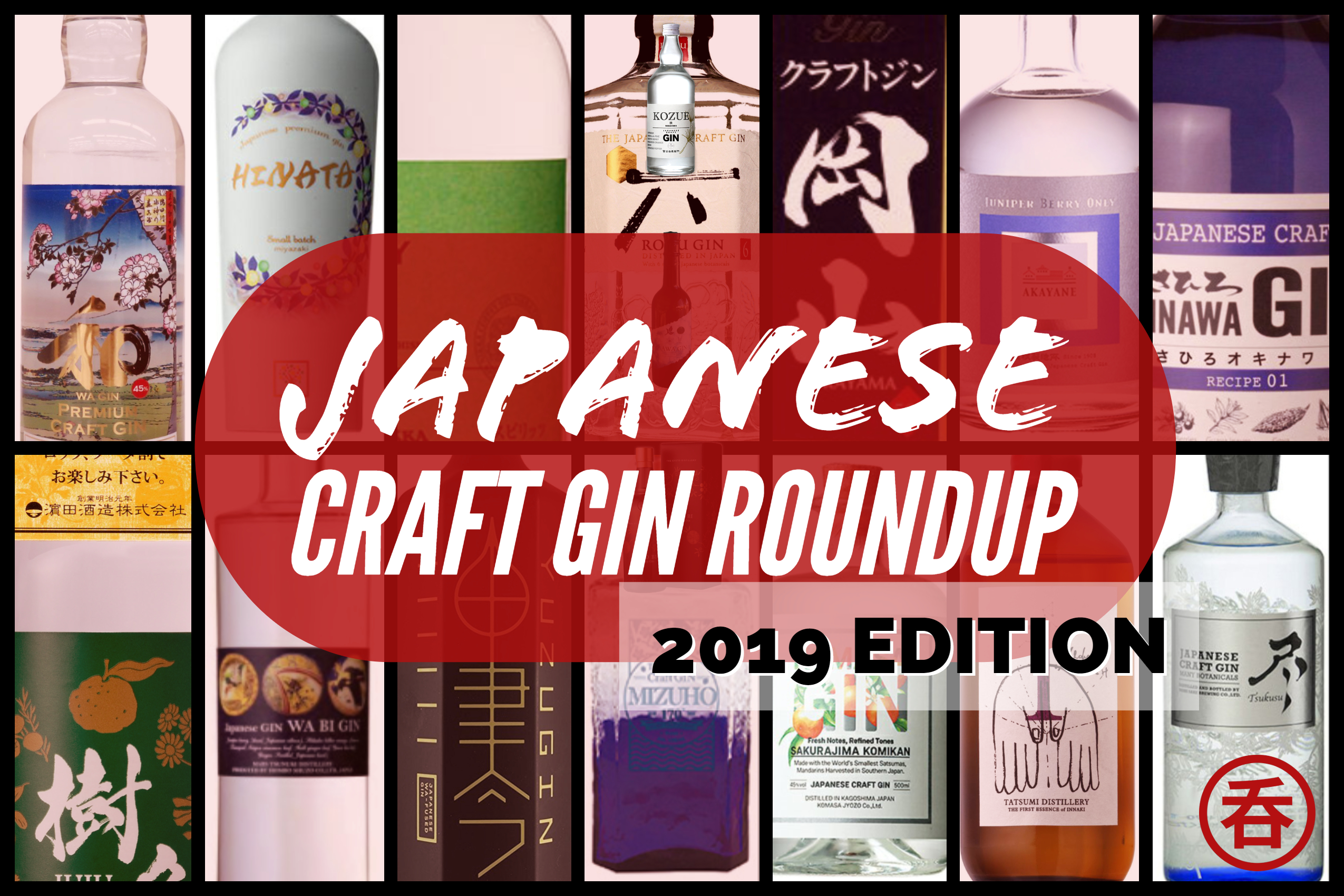The image is a horizontal, color illustration that features a black-outlined rectangle divided into 14 smaller rectangular sections, with each section displaying different bottles of gin. At the center of the image is a prominent red, pill-shaped oval containing the white text, "JAPANESE CRAFT GIN ROUNDUP" in all capital letters. Below and slightly to the right of this, the phrase "2019 EDITION" is displayed in black text, also in all capital letters, using a sun serif font. The bottles themselves showcase a variety of designs, ranging from clear glass to more opaque white and colored bottles. The labels, mostly in Japanese with some text too small to read clearly, include one labeled "Hinata." The background and bottle designs feature a mix of colors such as black, white, gray, brown, pink, purple, blue, orange, and red, indicating high-end brands with both floral and simple aesthetic styles. The overall theme of the image is to celebrate and rate different types of Japanese craft gin from the year 2019, highlighting their taste and overall drinking pleasure.